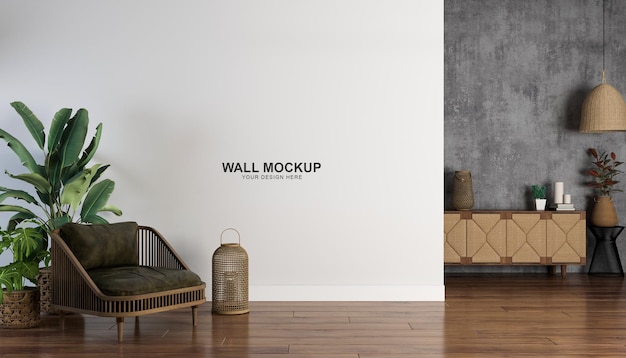This image captures a modern, intricately decorated room that features a prominent white wall which occupies about two-thirds from the left side. Centered on this wall, there’s black text reading "wall mockup, your design here," an invitation for customization. The wooden floor beneath showcases a light brown, neutral tone with a subtle shine, extending horizontally across the room.

On the left side of the room, situating in front of the white wall, there's a wooden armchair with dark green cushions, behind which stands a vibrant palm plant, adding a touch of nature to the space. Adjacent to the armchair is a brown couch with wooden legs and matching cushions, enhancing the cozy and warm ambiance of the room.

Further to the right of this seating arrangement, but still within the frame of the white wall, there is a wooden cabinet with a woven lamp, providing soft illumination, and a small clay pot with a green and brown plant. Behind these items, the space transitions into a gray wall which adds depth to the room's color palette.

The right-most section of the image features a cabinet that serves as a decorative focal point with an artfully placed light fixture hanging from the ceiling above. This beautifully balanced composition of furniture, nature elements, and thoughtful decor creates a welcoming and stylish environment, maintaining an inviting and modern vibe.